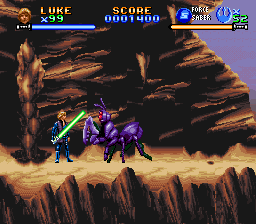In this color, computer-generated screenshot from the Super NES video game "Super Star Wars," Luke Skywalker, sporting his signature Return of the Jedi outfit with blue pants and a blue shirt, is captured mid-battle against a giant purple ant with red eyes on the edge of a cliff. Luke, wielding a green lightsaber, stands on a yellow trail set against a backdrop of brown rocks and a cave-like environment. The game interface is visible, with a widget in the top left corner displaying 'Luke,' alongside an image of a blonde-haired character, his full life indicated by a blue bar and the number 99. Centered at the top of the screen is the score, showing 1,400 in orange and blue numbers. On the right-hand side is the indicator 'Force Saber,' with an accompanying blue health bar and an orange life bar, showing full life. This detailed moment illustrates the intense action and vibrant graphics of this classic video game.